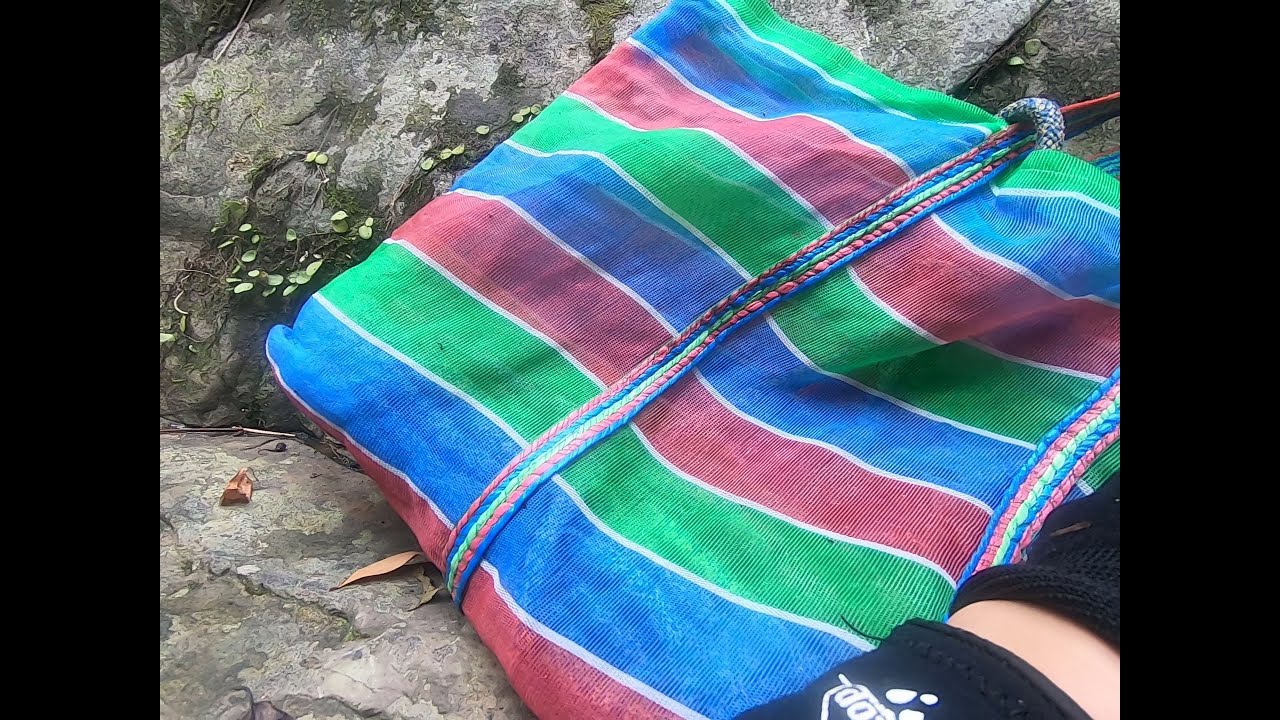In this bright outdoor scene, a large, striped bag or blanket is prominently featured against a backdrop of gray rocks adorned with green lichen, algae, and scattered dried leaves. This item, which has the appearance of a mesh or burlap material, is decorated with alternating stripes of red, blue, green, and thin white lines. The stripes run horizontally, while its braided handles, which have a rope-like texture, run perpendicular to them. The bag appears somewhat translucent. In the lower right corner of the image, part of a person is visible—possibly an arm or leg, clad in dark clothing, with a glimpse of skin and what seems to be a neoprene glove and a sweater. The setting suggests a rock climbing scenario, further emphasized by the rocky backdrop and the outdoor environment.